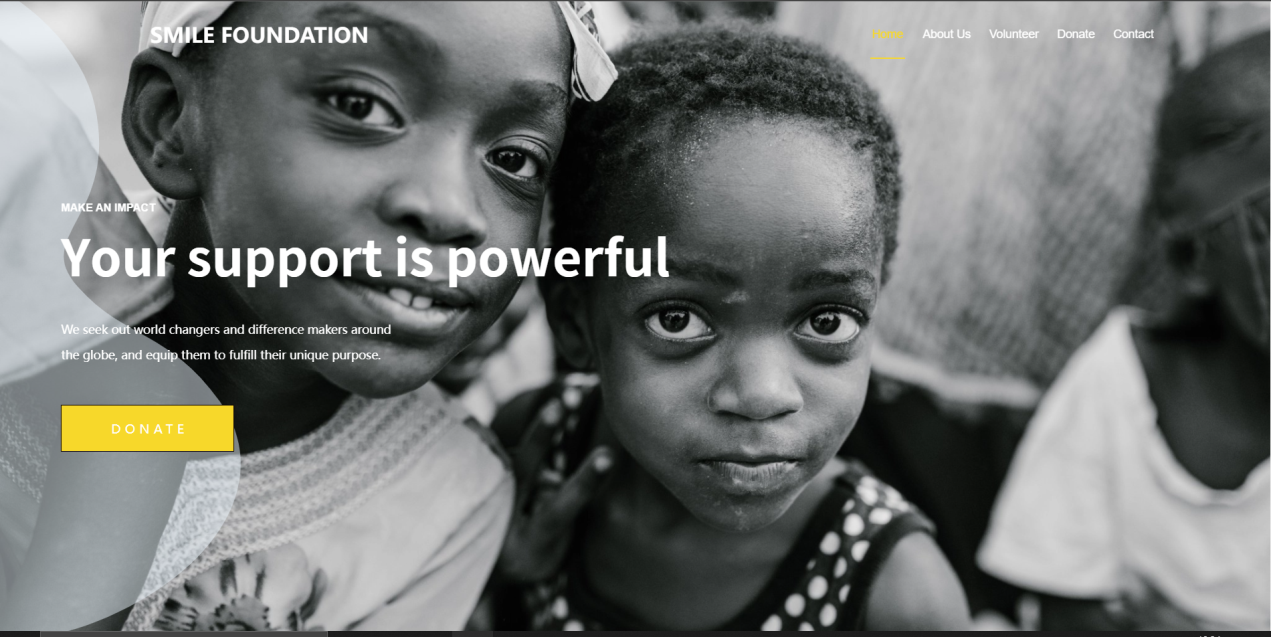This is a detailed screenshot of a web page from the Smile Foundation. The background of the page is a striking black and white photograph featuring two dark-skinned children who are gazing directly at the camera. The child on the left is smiling warmly, while the child on the right has a neutral expression. 

At the top of the page, a navigation bar is visible with menu options including "Home" (which is currently selected), "About Us," "Volunteer," "Donate," and "Contact." Below this, the text "Your support is powerful. Make an impact." is prominently displayed, followed by a mission statement: "We seek out world-changers and difference-makers around the globe and equip them to fulfill their unique purpose." 

A vivid yellow rectangle with the word "Donate" in white letters stands out, encouraging visitors to contribute. The overall layout of the image is notably wider than it is tall, ensuring a panoramic view that focuses solely on the children without any distractions from animals, birds, plants, flowers, trees, signs, billboards, flags, banners, automobiles, motorcycles, bicycles, airplanes, helicopters, or mountains.